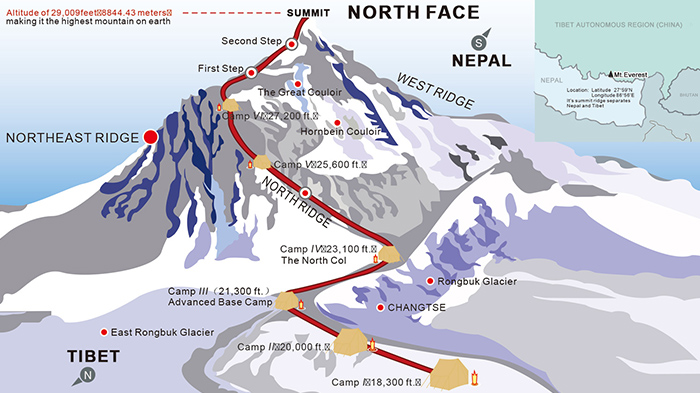The image is a detailed, annotated drawing of Mount Everest, set against a blue sky backdrop. The map highlights the Northeast Ridge and depicts various terrains including snowy white and gray sections. The summit is prominently labeled "Summit" at the very top, where it also says "North Face" and "Nepal" in black text. The elevation of 29,009 feet (8,848.43 meters) is marked in red text, emphasizing that it's the highest mountain on Earth.

A red path is illustrated, indicating the climbing route from the base to the summit. Key points along this path include "Second Step," "First Step," "Hornbane," "Colour," "North Ridge," "Advanced Base Camp," and several camps (Camp 1, Camp 2, Camp 3, Camp 4). The bottom-left corner of the map notes the location as "Tibet," while the upper-right includes an overlaid map labeling the broader region as "Tibet Autonomous Region, China," confirming the mountain's identity as Mount Everest.

This caption highlights the comprehensive nature of the map, showing both the specific climbing route and regional context.